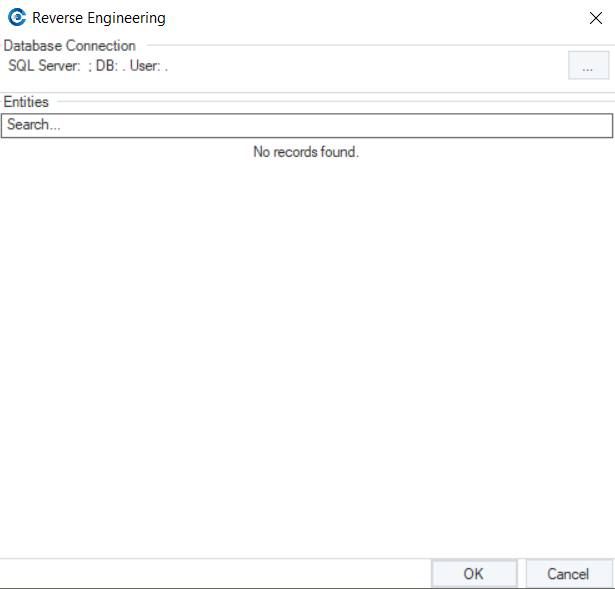**Caption:**

This is a rather basic website. In the top-left corner, there is a large "C" logo, nearly closed like a circle, containing a blue circle inside. The logo features a dark blue and light blue color scheme. To the right of the logo, in black text, it says "Reverse Engineering," and further to the right, there is a black "X."

Below this section, it reads "Database Connection" followed by a long, thin line. Underneath, there is text in which "SQL" is fully capitalized, followed by "Server" with a capitalized "S". It continues with "....DB" (DB in caps) followed by "..User" (User with a capitalized "U"). To the far right of this line, there is a dark gray rectangle containing three black ellipses.

A thin blue line follows this section, accompanied by black text that reads "ENTITIES", spaced out as "E N T I T I E S." Another thin blue line runs across right below this text.

Beneath these elements, there is a rectangular section extending from the left to the right with a bold black border around it. Inside, in black text, it says "Search..." Towards the center of this rectangle, it displays the text "No records found."

At the bottom of the page, there is a thin blue line followed by a thin black line. Between these lines, on the right-hand side, there are two mid-gray buttons: one labeled "OK" (with both the "O" and "K" capitalized) and the other labeled "Cancel" (with a capitalized "C").